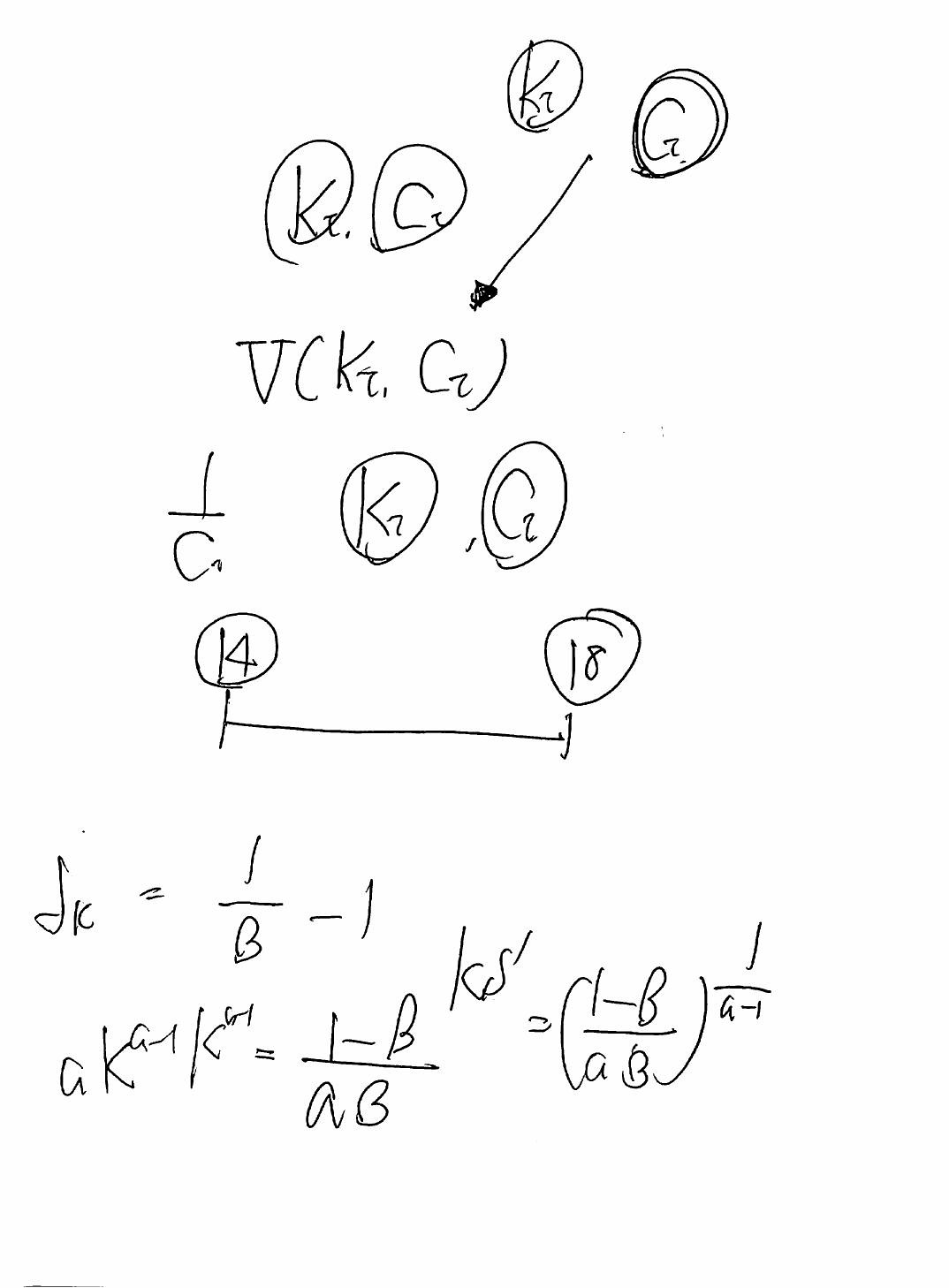**Detailed Caption:**

The image appears to be an intricate equation, possibly incorporating elements of both mathematics and chemistry, rendered in black writing on either white paper or a whiteboard. The layout is as follows:

- At the top left corner, there's a segment featuring "K2" enclosed in a circle.
- To its immediate right is "C2," also circled.
- Above this pair and slightly to the right, another "K2" and a "G" are each enclosed separately in circles.
- An arrow extends downward from the circled "K2" and "G", passing by the "KC" on the left, and points to "VCK2C2" with an inverted slash beneath it.
- Directly under this, there is a fraction "1 over CA" with "K2" and "C2" circled beneath it.
- Lower down, "14" is circled on the left, and "18" is circled towards the right.
- Both numbers are connected by lines that descend vertically before meeting at another horizontal line, forming a goalpost-like shape.
- Below this formation on the left side is a symbol that resembles a tangent sign, followed by the equation "K = 1 / (B - 1)".
- Beneath this equation is "aK" with a superscript "-1" on its right side, followed by "KG-1 = 1 - B / B".
- Slightly above and to the right of this segment is "KS1" with the equation in parentheses: "(1 - B) / (aB)" raised to the power of “1 / (a - 1)”.

This detailed depiction offers a clear view of the equation's structure and intricate connections.